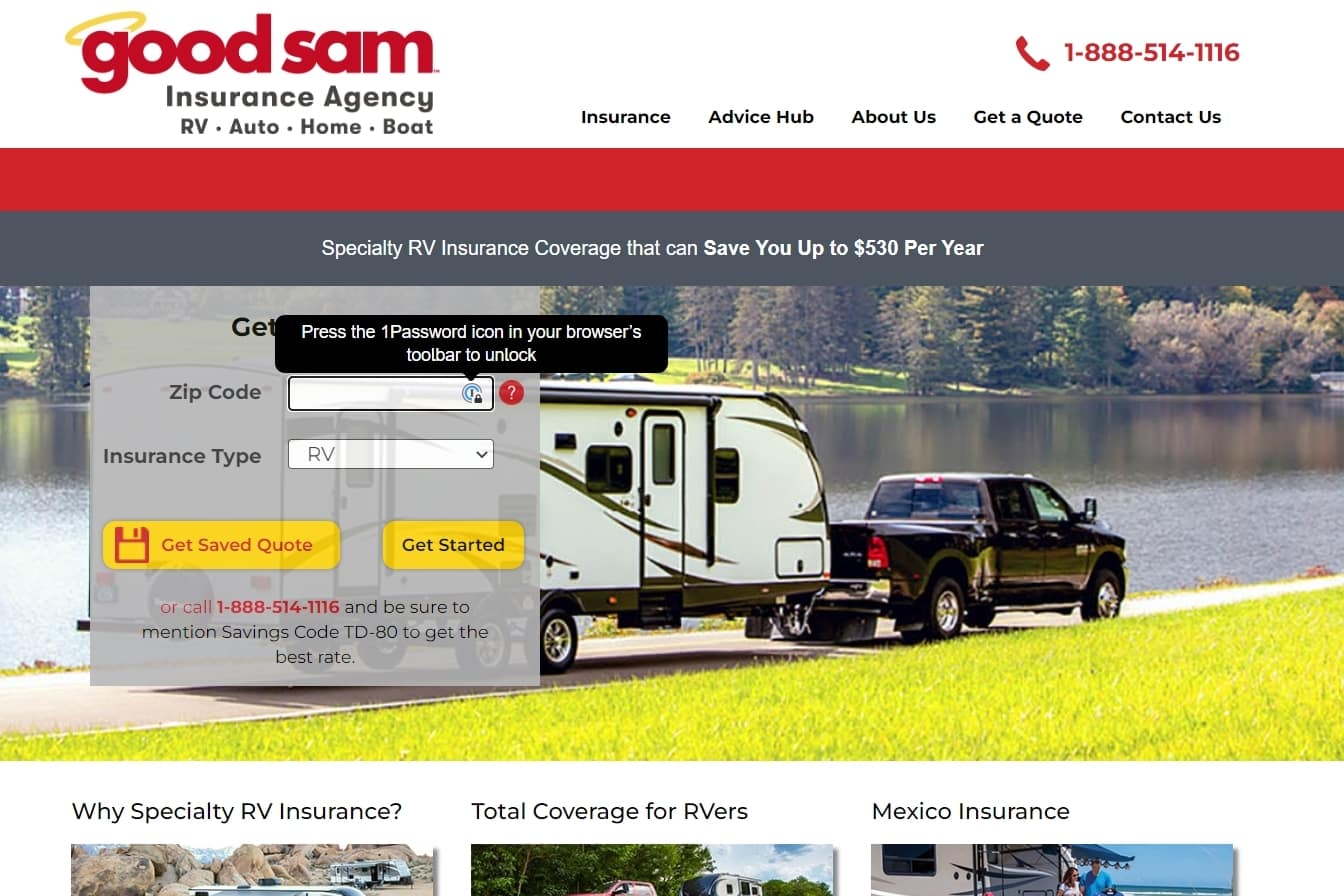The image is a screenshot of a web page for Good Sam Insurance Agency, prominently featuring the company’s logo in lowercase red letters with a yellow halo over the "G" in "Good." Adjacent to the logo is a red handset telephone icon beside the phone number, 1-888-514-1116. Underneath, "Insurance Agency" is displayed in a dark gray font, listing services for RV, auto, home, and boat insurance. 

At the top, there is a navigation bar with tabs in black text labeled: "Insurance," "Advice Hub," "About Us," "Get a Quote," and "Contact Us." Below the navigation bar, a red and gray banner with white text advertises specialty RV insurance coverage that can save customers up to $530 per year. The banner also features a "Get a Quote" pop-up option where users can enter their zip code and insurance type. Notably, there are two yellow buttons labeled "Get Quote" and "Get Started."

Centrally positioned in the webpage is a photo of a black truck towing a small fifth-wheel trailer, which is white and gray. The scene captures the vehicle towing the trailer alongside a large body of water, surrounded by trees and grassy terrain, emphasizing the outdoor adventure theme associated with RV usage.